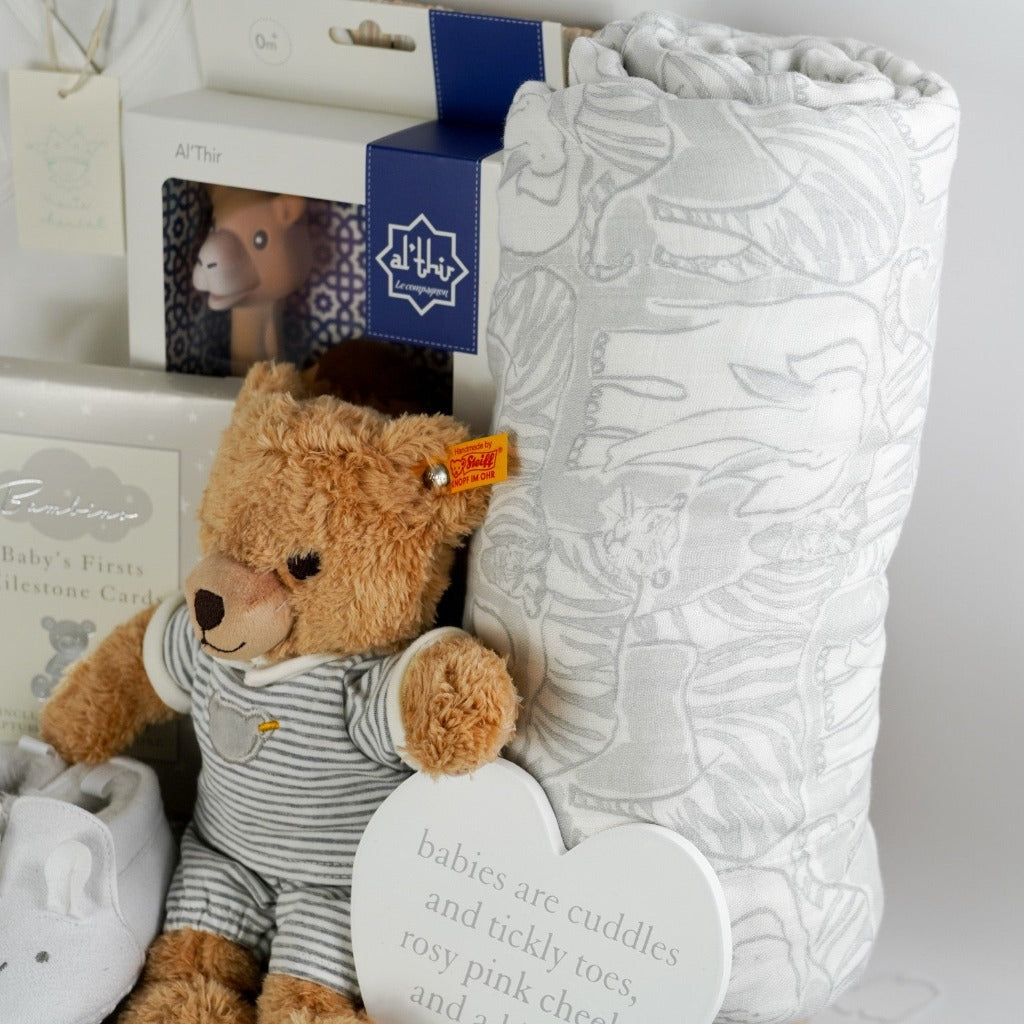This photograph depicts a collection of baby gifts arranged against a light gray background. Central to the image is a small, tan teddy bear dressed in a black and white striped shirt and shorts, complete with little slippers resembling mice. The bear also has a yellow tag on its left ear that reads "Handmade by Stuff." To the right of the bear, there is a neatly rolled blanket, which is gray and white and adorned with African animal patterns, including lions, elephants, and zebras.

In the foreground, a heart-shaped wooden plaque bears the partially visible text, "babies are cuddles and tickly toes, rosy pink cheeks." Positioned behind the teddy bear, a boxed toy featuring a brown animal with a long neck—possibly a giraffe or camel—labeled "Althier" inside a white box with a blue stripe on the right side. Lastly, on the left side of the image, a silver box is labeled "Baby's First Milestone Cards," featuring a silver bear icon below the text. This detailed arrangement suggests these items were carefully selected as gifts, likely for a baby's first birthday.